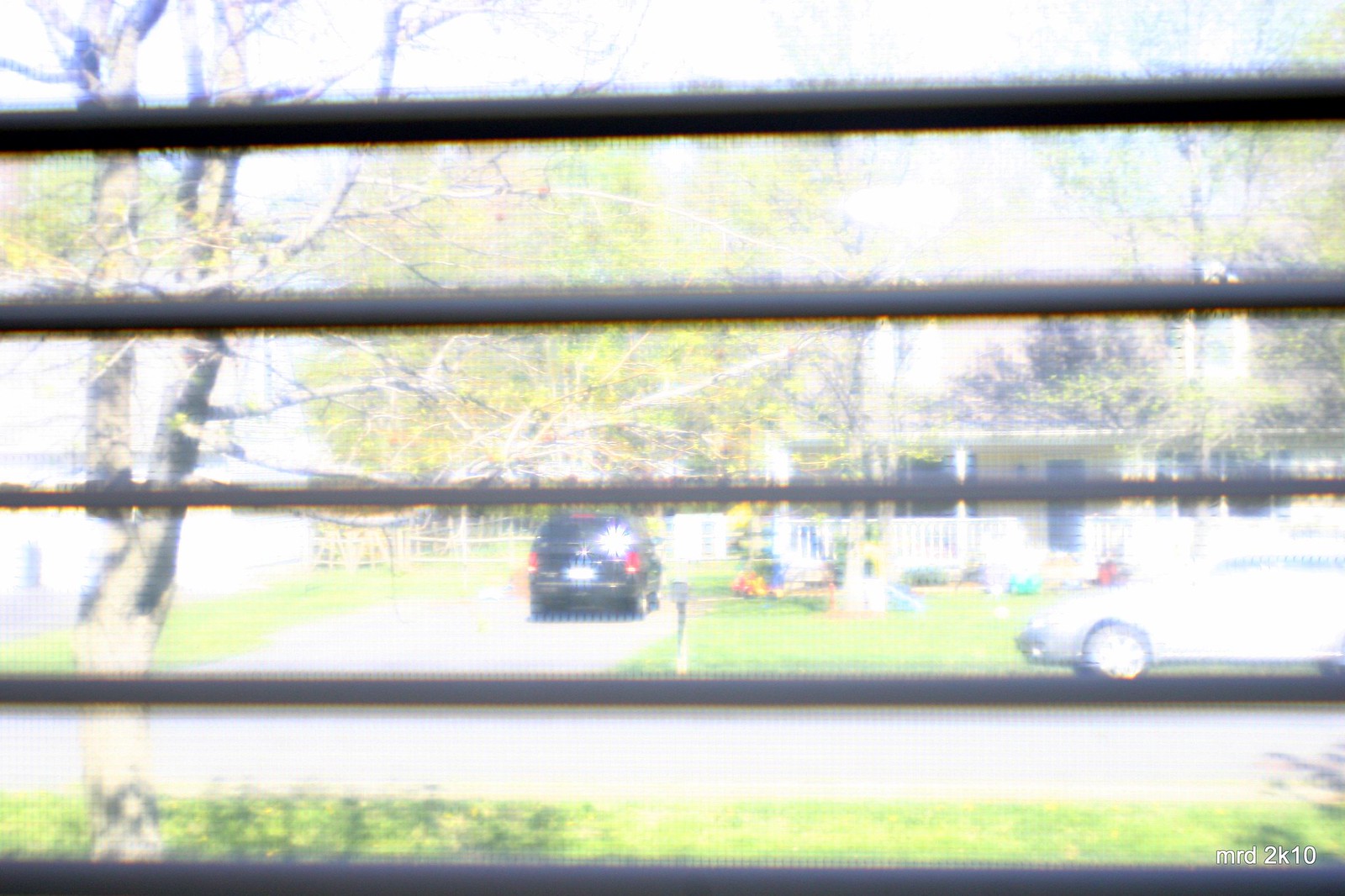A photograph captures the view from inside a house, looking out through a screened window. In the bottom right corner, white text reads "MRD2K10." The mesh screen overlay is visible, and five horizontal gray lines from the window blinds partially obscure the scene. Outside, a green lawn stretches across the street, where a yellow house with a gray roof sits, surrounded by a white rail fence. To the left, the trunk of a brown tree is seen, while on the street, a silver car is parked. Additionally, a black car is in the driveway of the house across the street, near a small brown and gray mailbox.